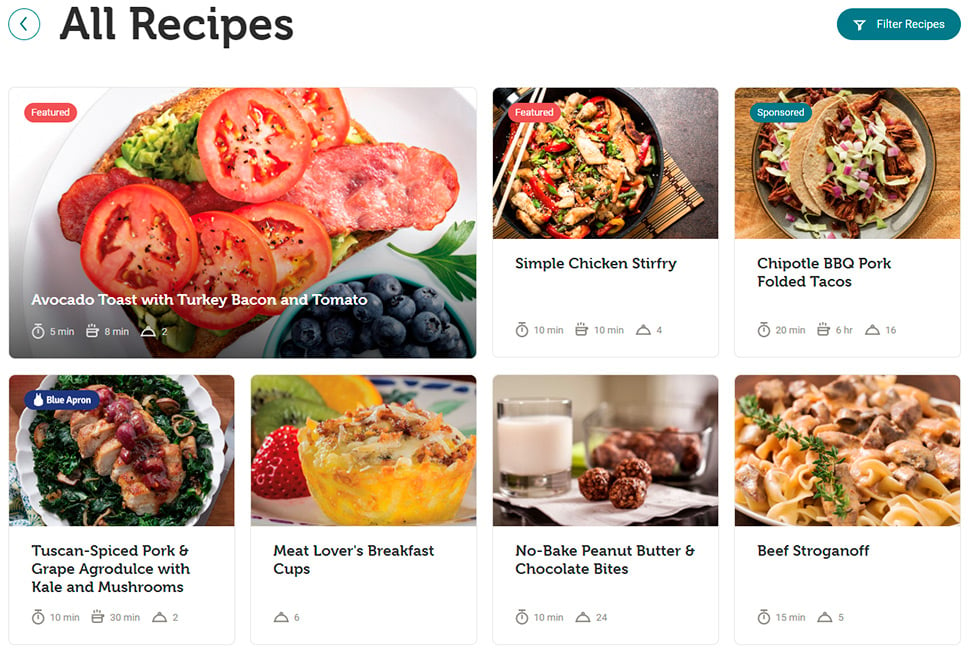This image is a screenshot from a website dedicated to recipes. The top portion features a navigation bar with a circular back button on the left, pointing to the left, next to the title "All Recipes." To the far right of this bar, there is an option labeled "Filter Recipes" highlighted in a greenish-teal color.

Directly below this bar, there's a prominently featured section with a red oval label saying "Featured." Below this label is a recipe titled "Avocado Toast with Turkey Bacon and Tomato," accompanied by a vibrant image. The image showcases the avocado toast, with a generous spread of smashed avocado, topped with turkey bacon and slices of tomato, surrounded by fresh blueberries.

To the right of this featured recipe, there are additional recipe options displayed in individual boxes. The first box highlights a "Simple Chicken Stir Fry," stating that it only takes 10 minutes to prepare. Next to it, there is a recipe for "Chipotle BBQ Pork Folded Tacos," which takes 20 minutes to make, along with an enticing picture of the dish.

Further down the page, the image reveals a variety of other recipes, including "Tuscan Spiced Pork," "Meat Lovers Breakfast," "No Bake Peanut Butter and Chocolate Bites," and "Beef Stroganoff." Each recipe is visually represented with its respective image and preparation time clearly indicated in its description.